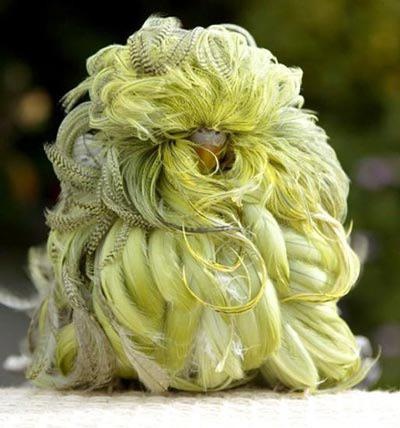This image showcases a peculiar and intriguing figure that could easily captivate and confuse an observer. At the center, there appears to be a small doll, reminiscent of the trolls popularized in the 1980s and 90s. This particular figure is engulfed in an extraordinary mass of what seems to be its hair. The hair, uncut and unkempt, has seemingly grown uninterrupted since the doll's creation, resulting in a sprawling and intricate coil that envelops its entire body.

The hair's dominant color is a striking yellow, interspersed with white patterns that add to the complexity and uniqueness of the visual. The material of the hair presents a texture that is both unusual and captivating, making it stand out. Despite its unconventional appearance, the figure does not invoke a sense of fear but rather a sense of wonder and curiosity.

This piece could be interpreted as an artistic statement on natural growth or perhaps an exploration of abandonment and neglect. The intricate details and the sheer volume of hair invite viewers to take a closer look and ponder the story behind this creation. It is a unique and odd figure that undoubtedly prompts a second glance and a thoughtful contemplation.